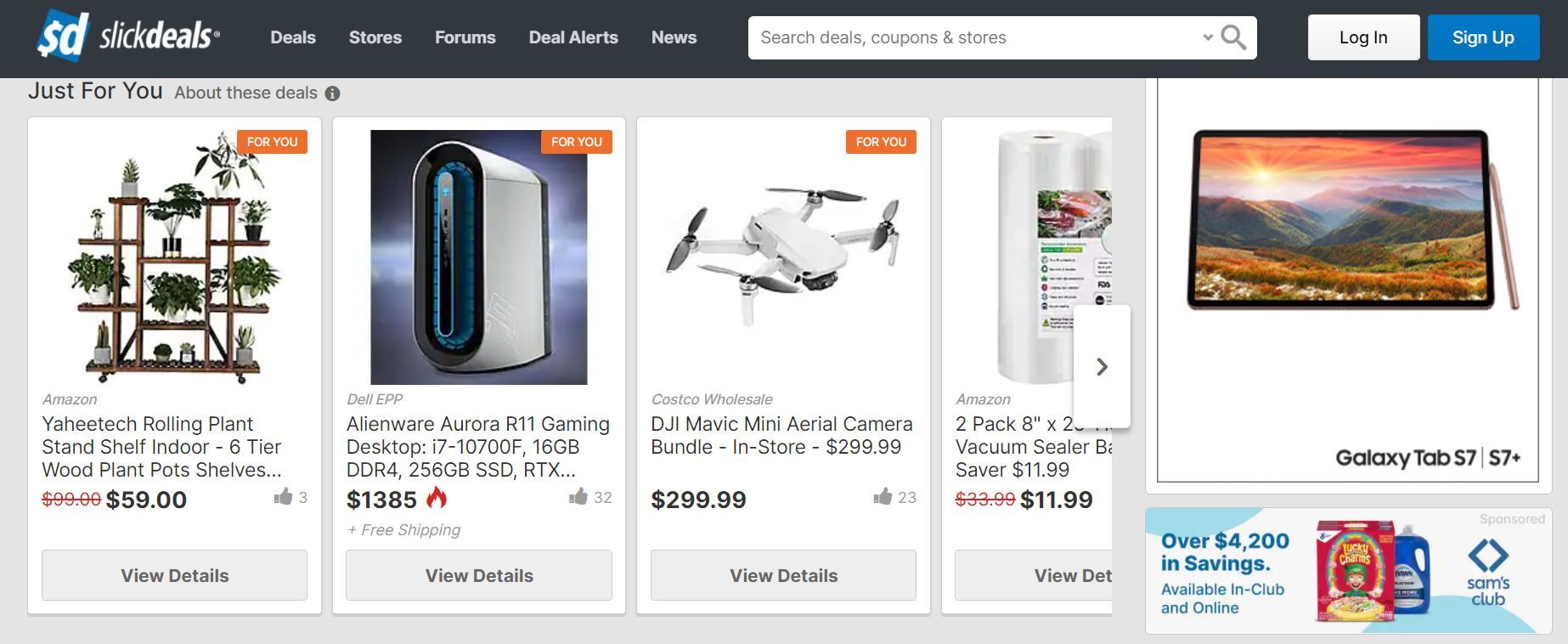This is a detailed screenshot of a search results product page from a website. At the top, there's a dark gray header featuring a logo on the left. The logo consists of a slightly rotated blue square with lowercase white letters "SD" on it, where the "S" is styled with lines extending from its top and bottom, resembling a dollar sign. To the right of the logo, the text "SLICK DEALS" is displayed in italicized white letters. Following this, there are several navigation sections in white text labeled as "DEALS," "STORES," "FORUMS," "DEAL ALERTS," and "NEWS." To the right of these sections, there's a white search bar with light gray placeholder text that reads "SEARCH DEALS, COUPONS, AND STORES," justified to the left. Adjacent to the search bar, a gray arrow points downward, and to its right, a gray magnifying glass icon signifies the search function.

On the far right of the header, there's a white button with gray text that reads "LOGIN," and further to the right, separated by a small gap, there's a blue button with white text that says "SIGN UP." 

Below the header is the product results page, organized with two advertisements on the right and a display of product listings on the left. The product listings are presented in panes with a white background. Each pane features a gray button at the bottom with the text "VIEW DETAILS" in the center. The screenshot shows three complete product panes and half of a fourth, which is partially cut off by the light gray background. Overlaid on the right side of the half-pane is a white rectangle containing a gray arrow pointing to the right, indicating more results.

Each product listing includes a picture and an orange rectangle in the top right corner displaying white text that reads "FOR YOU." Below the picture, the retailer's name is shown in italicized text, followed by the product name in large sans-serif text. The product price is displayed in black beneath the product name, along with other relevant details.